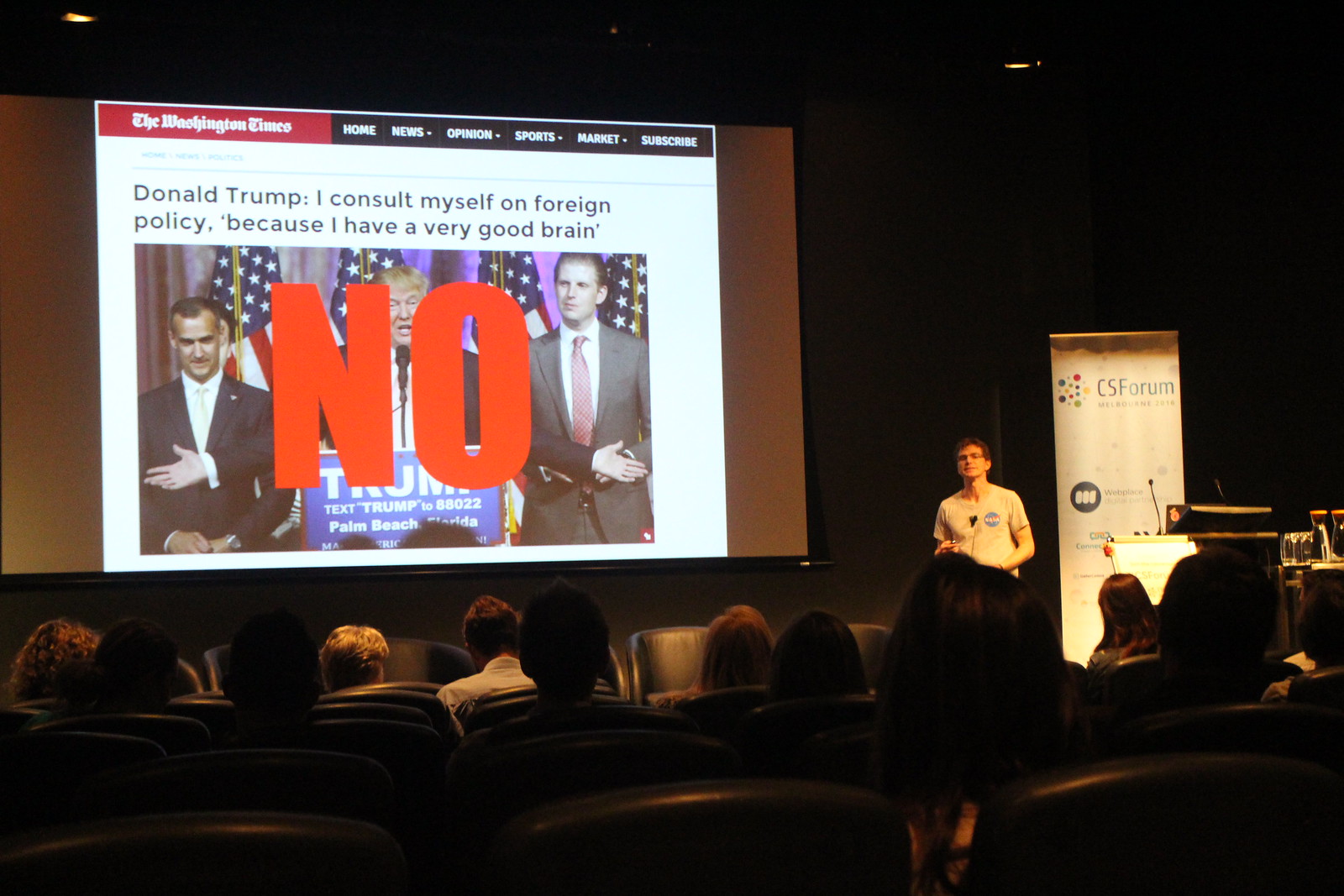The photograph captures the interior of an auditorium during a presentation. A man stands to the right, wearing a t-shirt and positioned next to an illuminated overhead projector, which displays an image on a screen. The projected content appears to be a news article from the Washington Times website, identified by the headings "Home," "News," "Opinion," "Sports," and "Subscribe." Prominently displayed on the screen is a quote attributed to Donald Trump, stating, "I consult myself on foreign policy because I have a very good brain," accompanied by a large red "no" in the center. Below the quote is an image of Donald Trump flanked by two men, likely including his son. The classroom or auditorium is dimly lit, with two or three rows of students or audience members visible in the foreground, attentively observing the presentation in near darkness. The banner reading "CS Forum" is also noted near the speaker, adding context to the event.